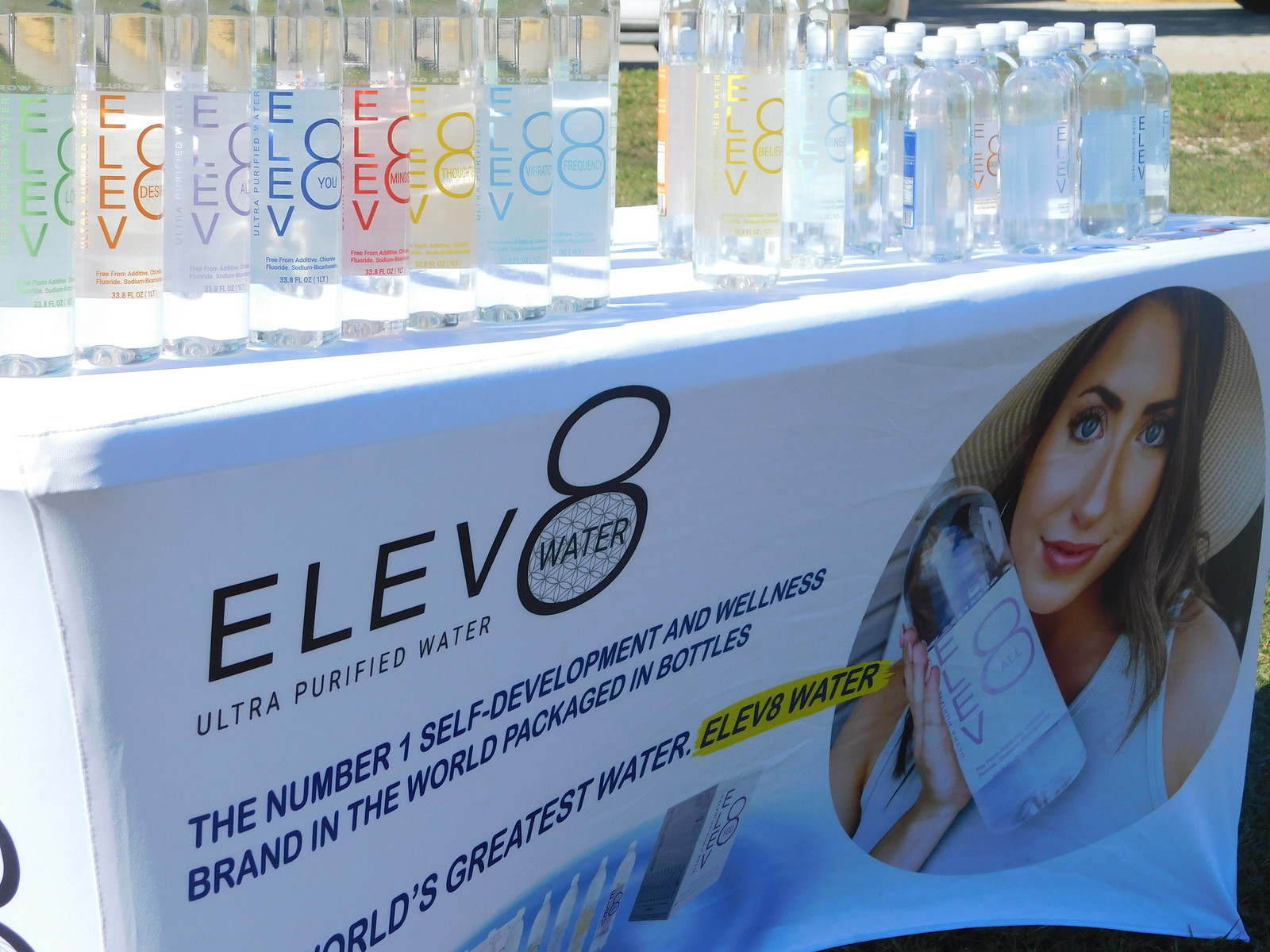The image appears to be an advertisement for Aleve 8 Ultra Purified Water, branded as the number one self-development and wellness water in the world. Central to the image is a white-clothed table set on a grassy background, suggesting an outdoor setting. Arrayed across the table are several bottles of Aleve 8 water in various colors indicating different flavors, such as green, orange, light blue, dark blue, red, and yellow. Each bottle is capped with a white top, reinforcing the brand's clean and pure aesthetic.

To the right side of the table, a beautifully pictured Caucasian woman, dressed in a white blouse that leaves her shoulders exposed, holds a large bottle of Aleve 8 water, gazing directly at the camera, giving the image a welcoming and engaging feel. The backdrop of the advertisement features a predominantly white poster with touches of blue, enhancing the purity and freshness associated with the brand. Prominently displayed on the tablecloth and the poster are the words "Aleve 8 Ultra Purified Water," "The number one self-development and wellness brand in the world," and "The world's greatest water."

Additionally, the tablecloth features the Elev 8 logo, which includes two circles stacked vertically. The top circle is plain white, while the bottom one contains black lettering spelling out "water" with decorative dots around it. The overall composition of the image is vibrant and visually appealing, reflecting the brand's emphasis on health, wellness, and high-quality hydration.